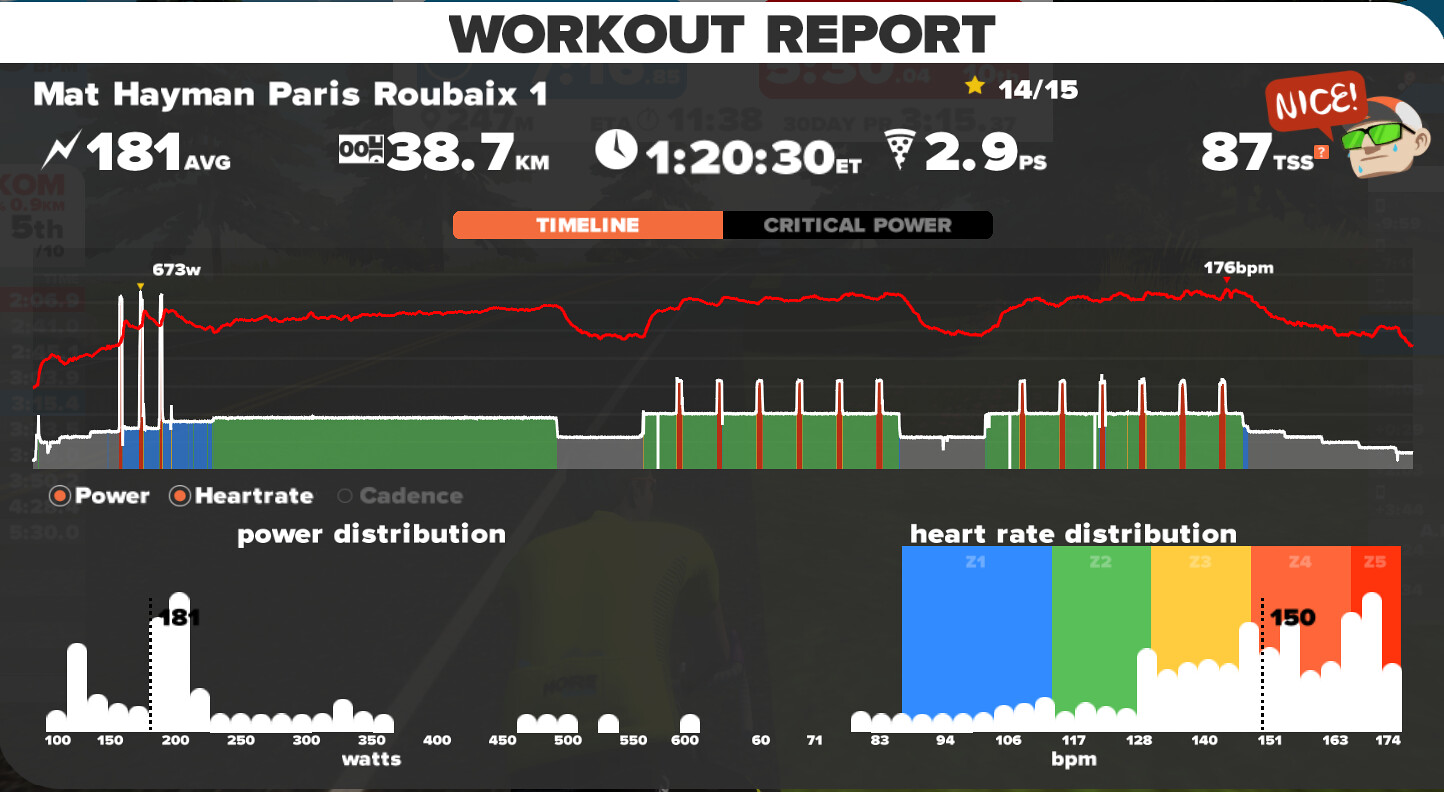This image is a detailed screenshot of a workout report for a cycling session by Matt Heyman at Paris-Roubaix 1. The report is more horizontally oriented. At the top left corner, the report title "Workout Report" is prominently displayed. Beneath it, the text "Matt Heyman Paris Roubaix 1" is accompanied by a yellow star and the stats "14 out of 15." Just below, the average power output is listed as "181 average."

To the right of the average power, the metrics continue with "38.7 kilometers," followed by the duration of "1 hour, 20 minutes, 30 seconds," and the unit "2.9 PS." Further to the right, the Training Stress Score (TSS) is shown as "87."

On the top right, there's an avatar of a man in a ball cap and green sunglasses with a speech bubble saying, "nice." 

In the center of the report, various graphs visually represent workout data, including power, heart rate, and power distribution metrics. The visualizations include horizontal green graphs with spiky vertical components. Below these, vertical white bars indicate watt data.

To the right side of the image, a multicolored graph in blue, green, yellow, orange, and red illustrates heart rate distribution, providing an in-depth view of the workout's intensity across various heart rate zones.